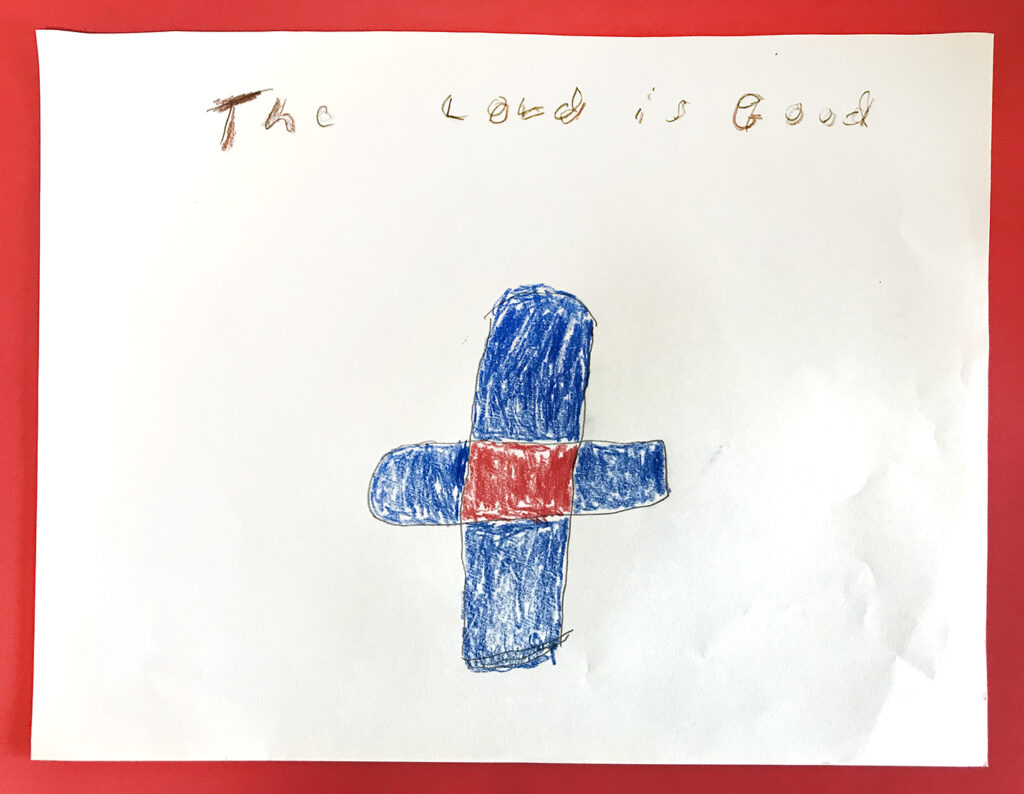This image is a child’s drawing, likely created during a Sunday school session. It features the phrase "The Lord is Good" prominently at the top, handwritten in a kid's script and initially drawn in pencil before being traced over with a brown crayon. The central element of the drawing is a blue cross with a red square in the middle, extending vertically on a plain white sheet of paper, which is bordered by a red frame. The cross’s distinct sections – top, sides, and bottom – are colored blue, while its center is red, giving it a somewhat band-aid-like appearance. The paper appears slightly wrinkled, hinting that the child may have crumpled or squeezed it while drawing. The overall image exudes the raw and earnest creativity typical of a young artist’s work.